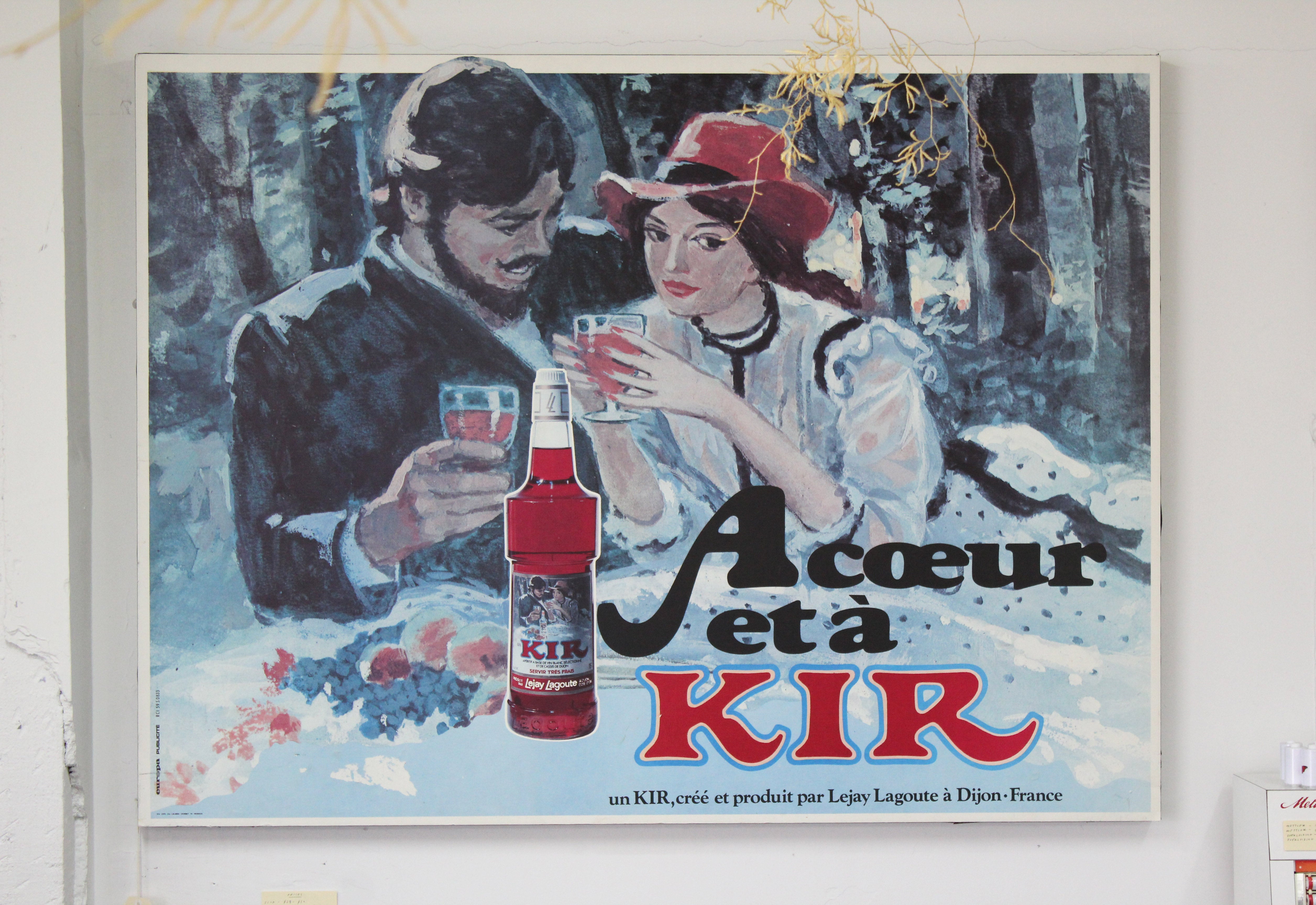The image depicts a vintage-style poster mounted on a white, slightly cracked wall. The poster features an intricately illustrated couple enjoying a drink outdoors in a snowy wilderness with tall, gray trees. The man, dressed in a black suit and sporting a beard, gazes lovingly at the woman, who wears a red bonnet and a lacy white frock with black trim. Both are holding glasses filled with a red liquid labeled "A Cure et a Care," with "A Cure et a" written in black and "Care" in red. The central bottle is a red liquid with a white cap. Additional French text at the bottom reads "Un Cure Cure et Produite par les Gers. La Goutte et Dijon France." The fond nostalgic ambiance is heightened by the depiction of the couple nestled cheerfully in the snow, the man with his arm around the woman, encapsulating a moment of shared warmth and joy.